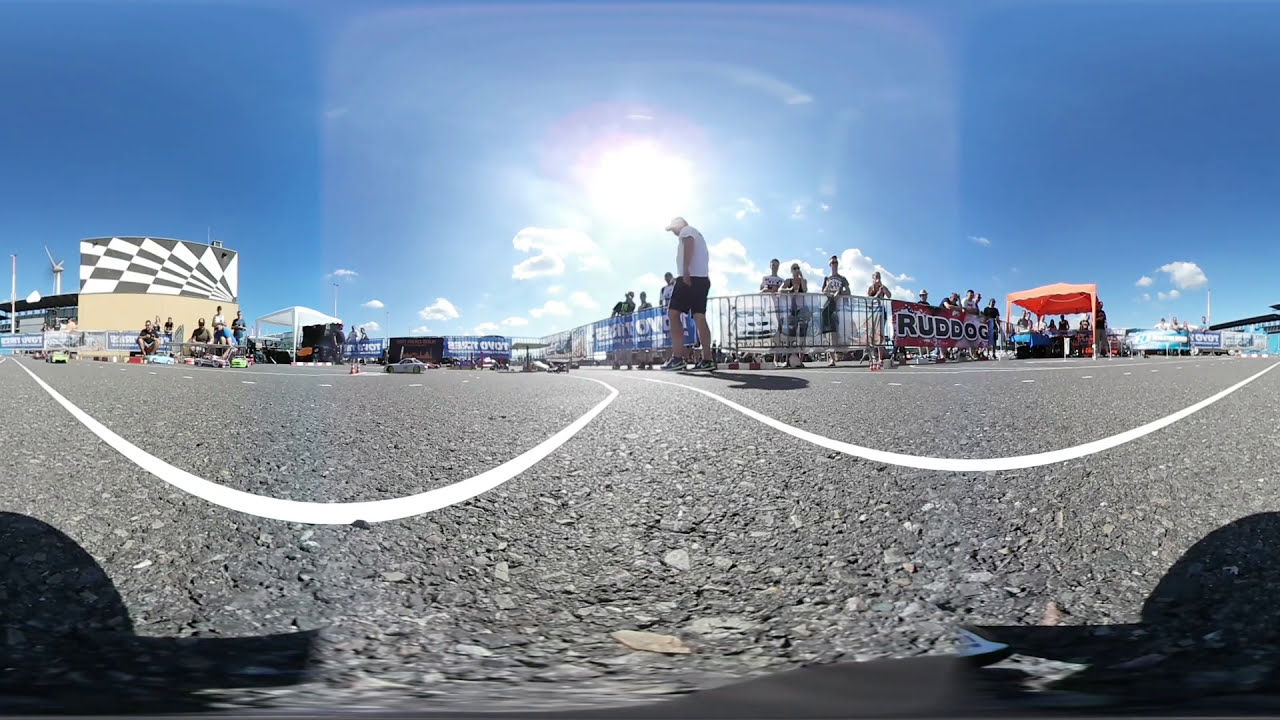The outdoor image, captured during the daytime, features a rocky, gravelly paved ground in the foreground, with noticeable bubble-like shadowing on the left and right sides. The background is dominated by a vivid blue sky with scattered, low-hanging clouds and a bright white sun in the upper half of the frame. The horizon line, where the sky meets the ground, reveals a tan building on the left with a prominent black-and-white checkered sign on top. A row of portable fencing stretches from left to right, displaying various banners, including one blue with white print, another red with black print reading "Red Dog, R-U-D D-O-G". An orange canopy tent is situated on the right side. Behind the fence, a crowd of predominantly male spectators is visible, with one man in a white t-shirt and black shorts walking in front of the fence. The foreground also features a section of a black-top surface with white lines, suggesting a remote control car racing track. The image exhibits a lens-altered effect, resulting in a bubbled distortion, particularly around the fence and gravel pavement, adding a dynamic perspective to the scene.